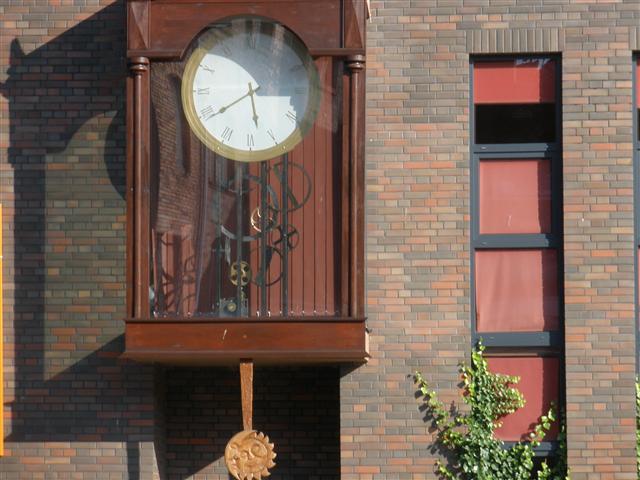The image depicts the exterior of a building adorned with multicolored bricks varying from grayish-brown taupe to vibrant orange-red. Bathing in the sunlight, the structure's facade includes a large, prominent grandfather clock. The clock, a striking feature in the image, showcases a pendulum shaped like a crescent moon and a sun, both with closed eyes as if in a serene embrace. Crafted from a lighter wood, the pendulum contrasts with the mahogany brown body of the clock. The clock face is framed with gold trim and features Roman numerals. The transparent casing of the clock reveals intricate black metal components, including various gears and wheels. Additionally, a vine ascends along the side of the building, winding around a vertical row of small square windows shaded in red, adding a touch of nature to the architectural scene.